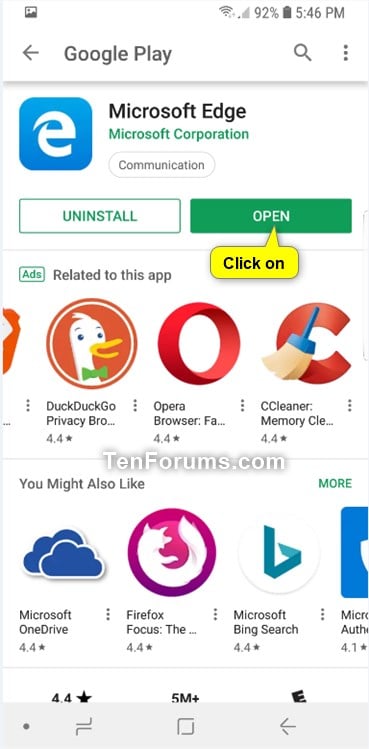This image appears to be a screenshot from an Android phone, showcasing the Google Play Store interface. At the top of the screen, the status bar displays essential information: the Wi-Fi signal icon, the cellular network bars, a battery level at 92%, and the time, 5:46 PM. Directly below the status bar, the heading "Google Play" is positioned with a back arrow to the left, a search bar in the middle, and a three-dot menu icon to the right.

The main focus of the screenshot is on the Microsoft Edge app page within the Google Play Store. The app is represented by a blue icon featuring a stylized "E." Below the app name "Microsoft Edge," the developer is identified as "Microsoft Corporation" under the Communication category. Two prominent buttons are displayed: an "Uninstall" button in white with a green outline and an "Open" button filled in green with white text.

Further down, there are advertisements for related apps, including DuckDuckGo Privacy Browser, Opera Browser, and CCleaner Memory Cleaner. Following the ads, there is a section titled "You Might Also Like," featuring suggestions such as Microsoft OneDrive, Firefox Focus, and Microsoft Bing Search, depicted with their respective icons.

At the very bottom of the screen, the Android navigation bar is visible, showing the home button, a multi-tasking icon (a square), and a back arrow to the left. Additionally, a watermark with the text "tenforums.com" is faintly visible, suggesting the source of the image.